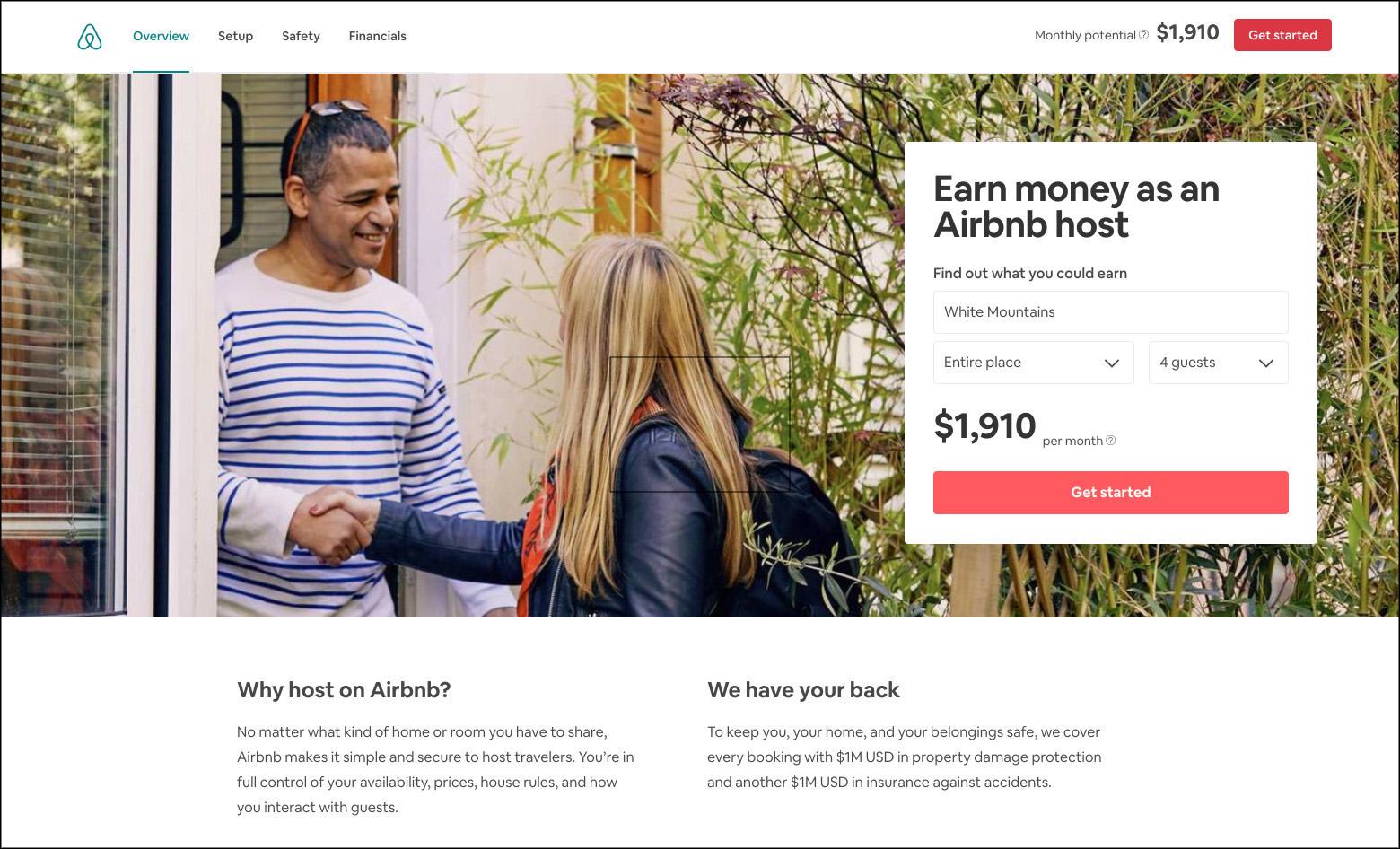This webpage showcases an enticing opportunity to become an Airbnb host. At the very top, the navigation menu includes links labeled "Overview," "Setup," "Safety," and "Financials" for easy access. In the top right corner, there is a highlighted potential monthly earning of $1,910 for hosts, and a call-to-action button encouraging users to "Get Started" to "Earn money as an Airbnb host" and "Find out what you could earn."

The main image features a serene scene set in the White Mountains, depicting an entire place available for rent that accommodates up to 4 guests. In the foreground, a man and a woman are seen shaking hands amidst a backdrop of greenery, including trees and plants.

The accompanying text invites prospective hosts to consider why they should host on Airbnb, emphasizing the simplicity and security of the platform. It assures hosts that they remain in full control of their property's availability, pricing, house rules, and guest interactions. Additionally, Airbnb offers robust protection for hosts, covering every booking with $1 million USD in property damage protection and another $1 million USD in insurance against incidents, ensuring peace of mind for property owners.